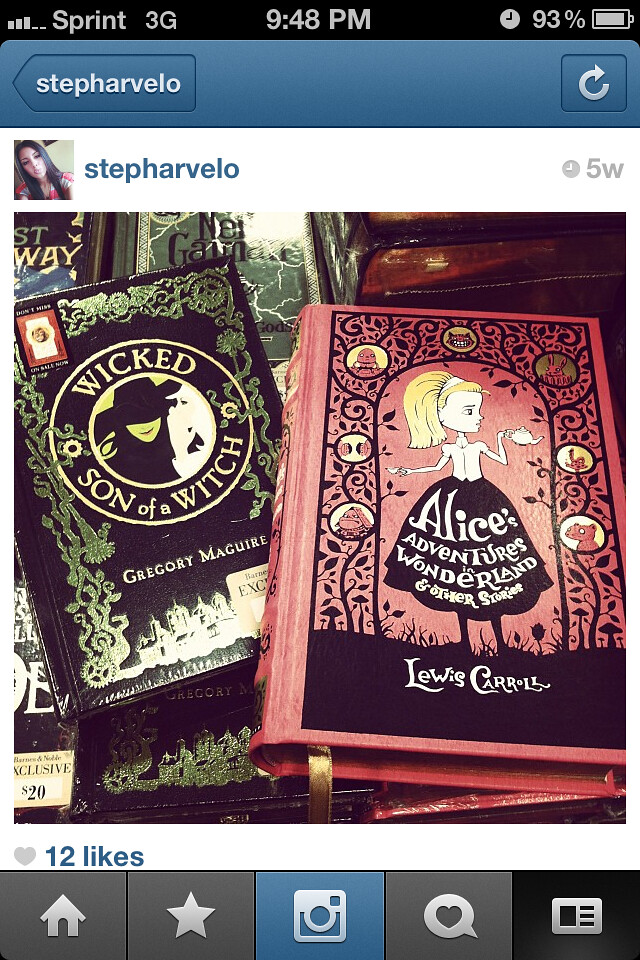The screenshot from an iPhone displays a social media post by user Steph Arvelo, taken at 9:48 p.m. with a 93% battery life, under a Sprint 3G network with three signal bars. The interface at the bottom includes five tabs: a home icon, a star, a camera, a speech bubble with a heart, and a contact card icon, set against a black background. 

The post features a blue rectangle banner at the top with Steph Arvelo’s name on the left and a refresh button on the right. Below this, her profile picture appears beside her name, indicating the post is 5 weeks old. The image in the post showcases two hardcover books: "Wicked: Son of a Witch" by Gregory Maguire, recognizable by its green trim and embossed gold cover with a green witch symbol, and "Alice’s Adventures in Wonderland and Other Stories" by Lewis Carroll, featuring iconic illustrations like the Cheshire Cat and a central image of Alice surrounded by vines and images of other characters. The post has received 12 likes.